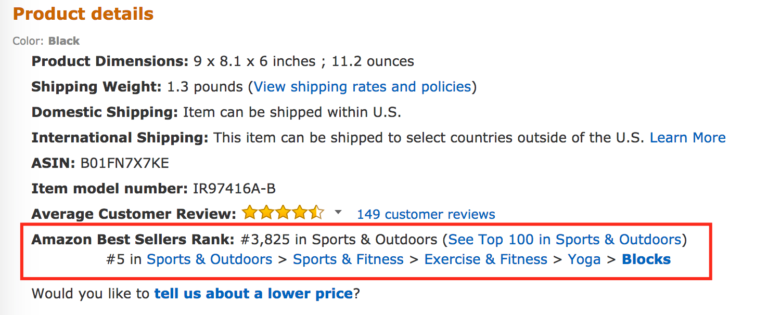Caption for the screenshot:

This image is a detailed screenshot from an e-commerce platform, likely either Amazon or eBay, showcasing the product details of a specific item. The title "Product Details" is prominently displayed in the top left-hand corner in a distinctive red-brown font. Below the title, a section bordered by a red rectangle highlights the Amazon Best Sellers Rank, indicating the item holds the position of number 3,825 in the Sports & Outdoors category and number 5 in the sub-category of Sports & Outdoors > Sports & Fitness > Exercise & Fitness > Yoga > Blocks. The background of the page is completely white, with all text being rendered in black. The detailed product description enumerates various important specifications including product dimensions, shipping weight, model number, and shipping information for both domestic and international orders. Additionally, it notes the item has garnered an impressive average customer review rating of 4.5 stars from a total of 149 customer reviews. At the bottom left-hand corner of the screenshot, there is an option saying, "Would you like to tell us about a lower price?"